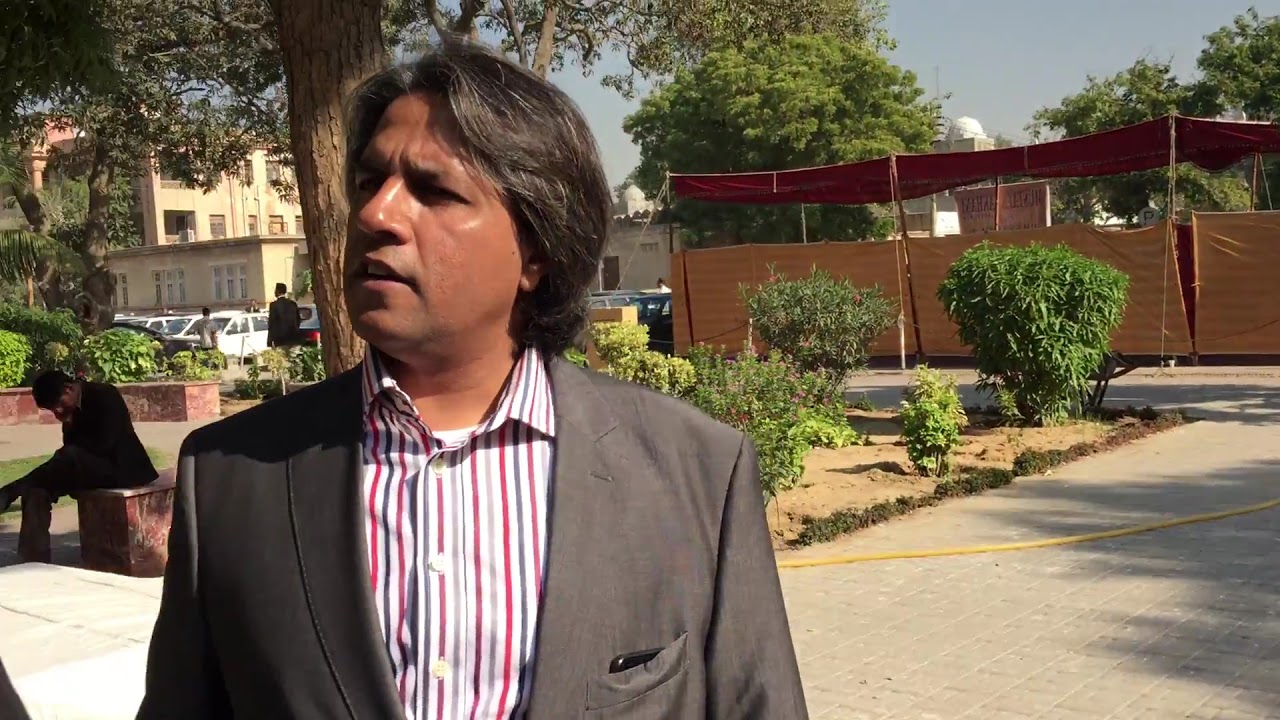The photograph features an older man with a rich brown complexion and slightly glossy skin, possibly multi-ethnic or Hispanic, standing outdoors in a park-like setting. He has dark charcoal gray hair and is dressed in a dark gray suit. Underneath, he wears a striped button-down shirt with red, light gray, and dark gray stripes, adorned with white buttons, and he has a cell phone visible in the left pocket of his suit. The man appears to be slightly confused, with furrowed eyebrows, and is looking off to the left side of the image.

In the background, a red tent with bright beige or brown walls stretches behind him, tied with ropes. There is also a large building painted in a light yellow mixed with orange color, visible in the upper left corner. The tree behind him has a brown trunk and green leaves, and adjacent bushes are also green. Additionally, there are some cars parked to the left of the tent, with a couple of people dispersed around the area. A stone bench beneath the tree hosts another person sitting, and there is another person walking in the background. A yellow hose runs along a sidewalk or walkway near some shrubbery and plants. The image captures a blend of urban and natural elements, depicting a multi-faceted outdoor scene.